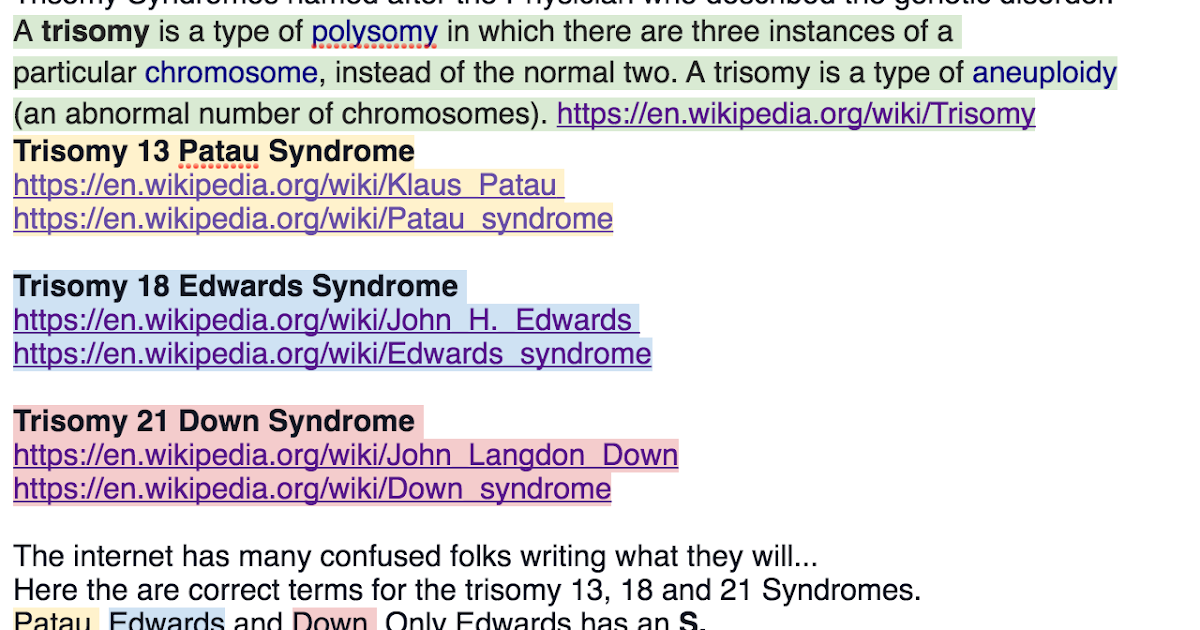This image displays research and citation information centered around various Trisomy conditions, presented on a white background with black text. The text features multiple sections, each highlighted in different colors to emphasize different parts of the content. Several sections also include Wikipedia links for further reference.

- The first paragraph, highlighted in light blue, explains that "A Trisomy is a type of polysomy in which there are three instances of a particular chromosome instead of the normal two. A Trisomy is a type of aneuploidy, an abnormal number of chromosomes." This section includes a hyperlink to the Wikipedia page for Trisomy.
  
- The next section, highlighted in peach, pertains to "Trisomy 13 Patau Syndrome" and includes two Wikipedia links: one for "Klaus Patau" and one for "Patau Syndrome."

- Following that, highlighted in medium blue, is information about "Trisomy 18 Edwards Syndrome," accompanied by two Wikipedia links, one for "John H. Edwards" and the other for "Edwards Syndrome."

- The section highlighted in light purple describes "Trisomy 21 Down Syndrome," and it also includes two Wikipedia links: one for "John Langdon Down" and one for "Down Syndrome."

- The final paragraph, in black text, states: "The internet has confused folks writing what they will. Here are the correct terms for the Trisomy 13, 18, and 21 syndromes. Patau, Edwards, and Down, only Edwards has an S."

This comprehensive layout provides detailed descriptions and corresponding sources for different types of Trisomy, making it a valuable reference for understanding these genetic conditions.